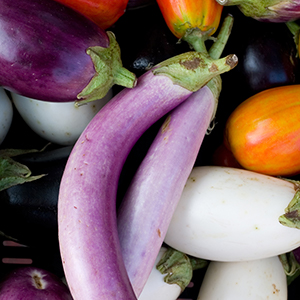The horizontally aligned, slightly blurry photograph showcases a vibrant assortment of vegetables, predominantly eggplants of various colors and shapes, likely from a food magazine or photography project. The image features narrow, curved Japanese eggplants, including a central one that is soft purple on the right with a white reflection and a green leaf-stem merging at the top. Adjacent is a darker eggplant slanting down from the top corner, with three leaves curled around the stem. Behind this darker one is another partially visible blackish-purple eggplant with additional white eggplants and a distinctive lavender one in the lower left corner. A cluster of three white eggplants is in the background, with partial views of a horizontally aligned one showing a leaf pointing left, another fatter one underneath, and a topside view with dry green leaves. Also visible are elongated orange-green tomatoes, more dark purple eggplants, and partial red tomatoes scattered amid the eggplants, adding to the colorful display. No full eggplant is entirely visible, but the array showcases the diversity within the eggplant family, complemented by hints of other vegetables like onions, and brings a lively, farm-fresh appeal to the image.